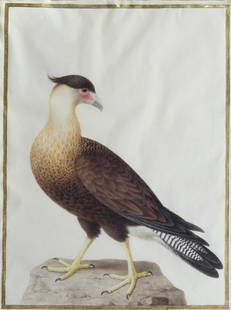This image depicts a detailed illustration of a hawk standing on a large, flat-topped, light-colored rock. The artwork is printed on cloth, enclosed within a very thin gold border that frames the light gray, almost white background. The hawk, facing left with its head turned to the right, showcases a striking combination of colors and textures. Its body features a mix of brown shades, with long, slender yellowish-white legs and feet ending in black claws. The bird’s tail feathers exhibit white and black pinstripes with black tips. The neck is a cream color that fades into tan as it connects to the darker-feathered chest and wings. The hawk's face is marked by a distinctive red area around the eyes, a gray curved beak, and a characteristic tuft of dark feathers atop its head, resembling an old man’s comb-over. The image size is relatively small, approximately one inch wide and no more than two inches tall, and contains slight wrinkles, adding to its textured, cloth-like appearance.